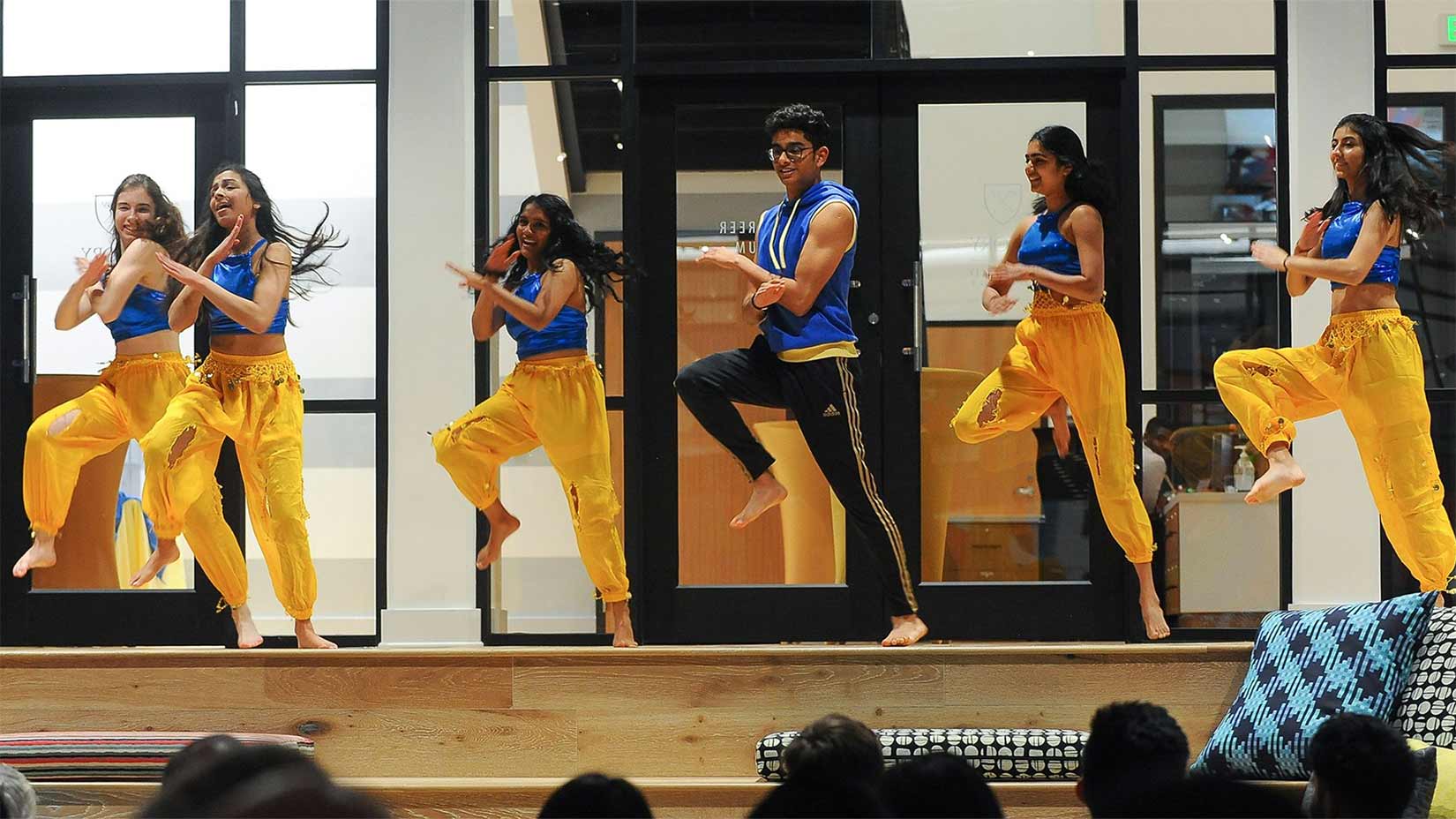This detailed image captures six dancers mid-performance on a wooden stage, evident by its light brown wood flooring. Five female dancers in yellow pants and blue crop tops surround a male dancer at the center, who stands out in black Adidas pants with yellow stripes and layers of a yellow sleeveless t-shirt under a blue sleeveless sweatshirt. Each dancer is dynamically posed with their right foot on the ground and their left foot raised. The backdrop consists of windows framed by black metal, revealing the architectural elegance with black-outlined white elements. The audience's presence is subtly indicated by the partial view of their heads at the bottom of the photo, suggesting they are adults with dark hair. Below the stage, large pillows and rolled-up yoga mats are visible, adding to the room's functional aesthetic.